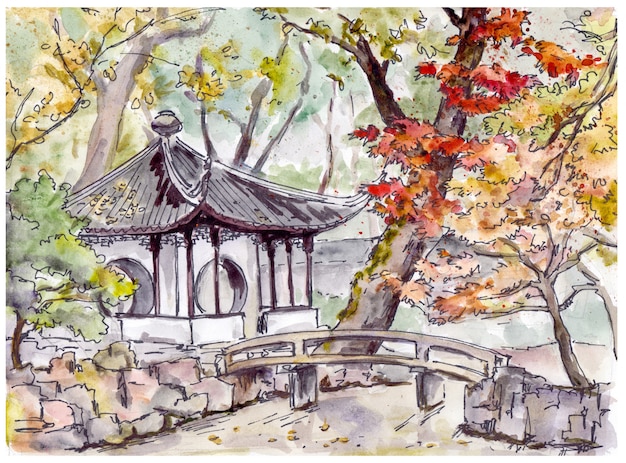In the watercolor painting, an elegant pagoda-style building with a white exterior and brown curved roof stands prominently amid a serene garden. The square structure features large, round entrances on the visible walls, complemented by a low stone wall that creates a peaceful walkway beneath the pagoda roof. In front of the structure, a stone pathway and a traditional arched bridge span a narrow canal, leading to the right side of the scene. Surrounding the bridge and building are an array of trees with trunks of brown swaying gently; their leaves display a beautiful fall palette of yellow, orange, red, and green, resembling maple leaves. One of these vibrant trees, positioned to the right of the bridge, provides dappled shade and enhances the tranquil atmosphere. The ground near the bridge is covered in gray stones and reflects the myriad colors of the foliage above. The setting appears to be a forest in autumn, with some leaves scattered in the water, capturing the essence of the season.